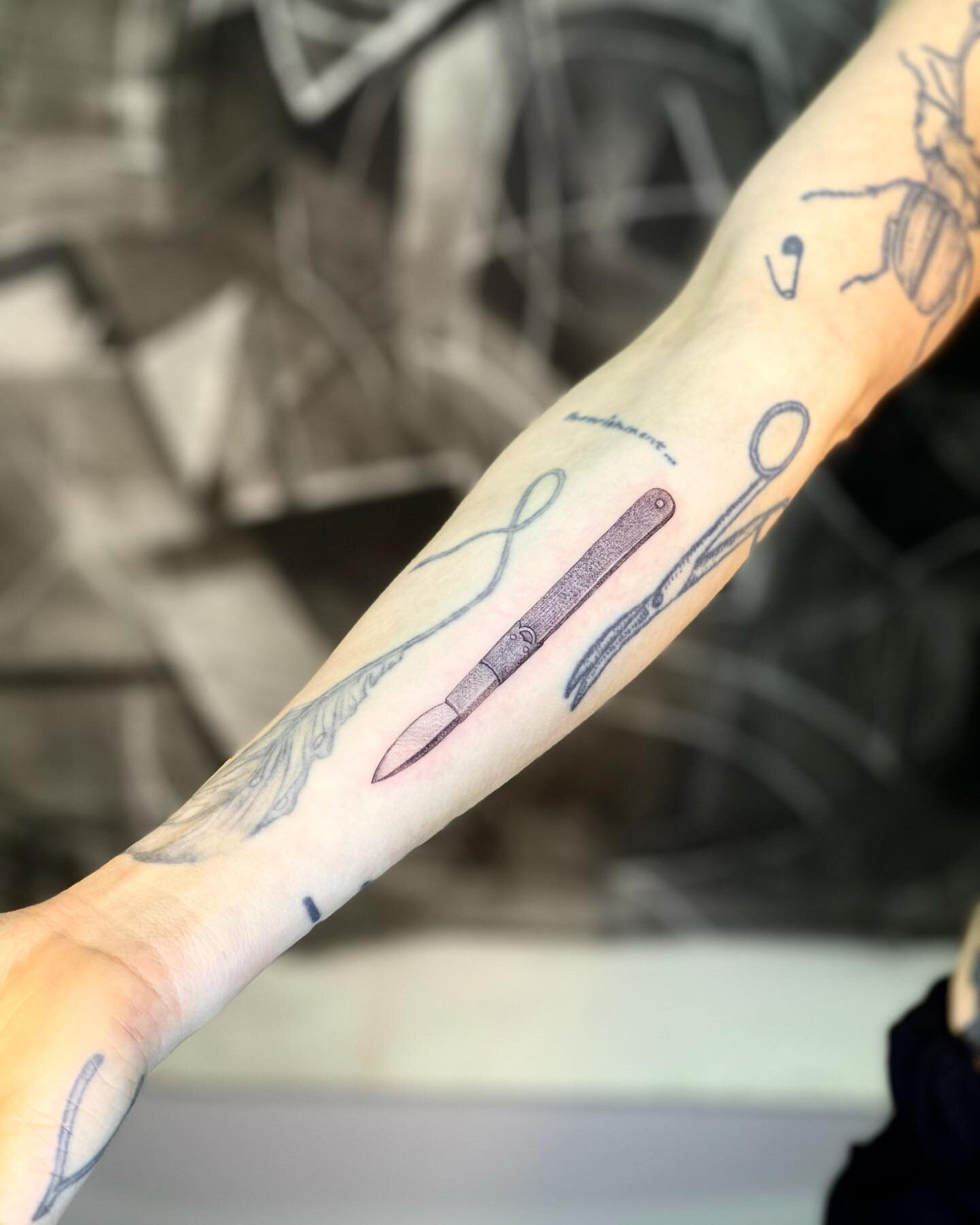The image depicts a person's pale, white arm adorned with numerous fine-line black ink tattoos, each representing different objects. From the top right of the arm cascading down to the hand, the tattoos include a linear design resembling a beetle at the upper portion. Below the beetle and slightly to the left is an open bobby pin. Around the elbow, a pair of scissors is prominently featured. Moving down towards the forearm, there is text in fine print that remains unreadable. Below the text, prominently displayed, is a vintage scalpel with a small blade and a wooden handle encased in a metal sheath. Adjacent to the scalpel, a leaf with a long string tied into a bow is visible. Further down near where the arm meets the hand, tattoos of a pair of tweezers or possibly a wishbone, and a pair of pliers are etched. The entire background is blurred, focusing attention solely on the detailed black ink artwork, revealing veins beneath the person's very pale skin.